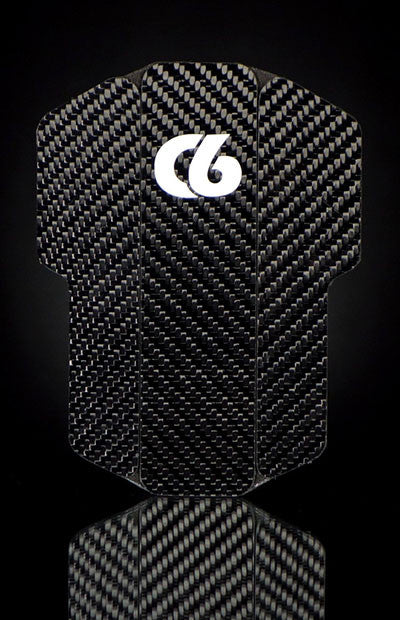The image features a textured, close-up view of a shin guard against a jet black background. The shin guard, centered within the frame, is crafted from 100% carbon fiber, showcasing a detailed weave pattern resembling a herringbone design. The gray fabric of the shin guard forms a shape akin to a mushroom, with a distinct head and shaft. The head measures roughly 2.5 to 3 inches in width, while the shaft is about 2 inches wide. At the top, the text "C6" stands out in white, with the letter 'C' artfully curling into the number '6'. Below this main section, the shin guard appears split, revealing a second piece that sits beneath the top part. This bottom section has a trapezoidal shape and features a similar yet slightly darker weave pattern with lines set at an angle.